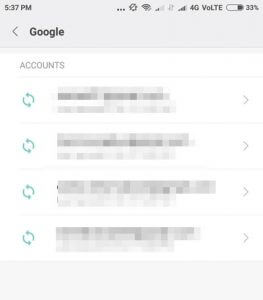The image appears to be a screenshot from a mobile phone's interface. At the top, there's a grey status bar. On the left, the time is displayed as "5:37 PM" in black font, while the right side features an ellipsis ("..."). Adjacent icons show the Wi-Fi signal, a pie chart icon, a 4G VOLTE indicator, and the battery level at 33%.

Below the status bar, to the left, there is a grey arrow pointing left. Next to it, in black font, is the word "Google." Beneath this, in grey font, the word "Accounts" is displayed, followed by a grey dividing line.

The main content area features four identical rows. Each row contains a green circular arrow icon, composed of two arrows circling each other, indicating synchronization or refreshing. These icons are slightly pixelated and have a grey arrow pointing downward next to each. These rows are separated by grey dividing lines.

At the bottom of the main content area, there is an empty grey box with no content inside.